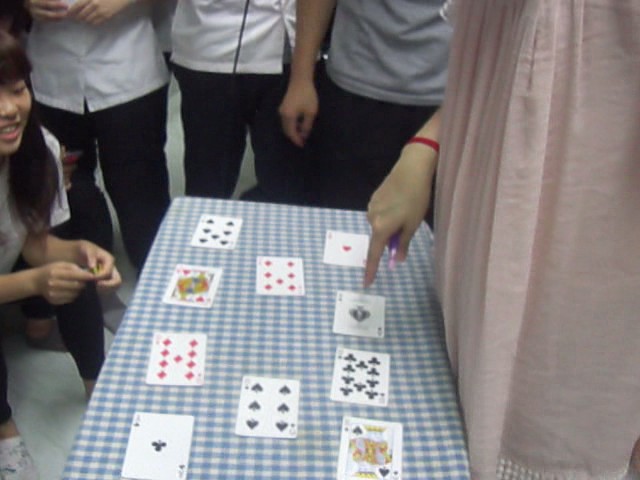In the image, a group of people is gathered around a table that resembles one used for card games. They seem to be engaged in the activity, with particular attention directed at the cards laid out on the table. A specific individual on the right, distinguished by a red wristband and dressed in a pink skirt or dress, is pointing at a card. 

Behind this person, other participants, possibly students, are present in black pants and white and gray shirts, standing with their hands by their sides. Toward the left, a girl is kneeling with her hands clasped together. She has long black hair, wears black pants, and a white shirt.

The table itself has a blue and white pattern draped over it. Several cards are spread out in distinct positions: 

- In the bottom-left corner, there is an Ace of Clubs.
- Directly above it, there is a card from the diamonds suit, followed by a face card from the diamonds suit.
- Above this, another card from the clubs suit is partially visible but blurry.
- In the middle row, there is another card from the clubs suit.
- At the top, there is a card from the diamonds suit.
- In the bottom-right corner, a King of Spades is visible.
- There is another clubs card beside it, and above those cards lie an Ace of Spades and an Ace of Hearts, all face up.

The scene is charged with the energy of a card game, with various participants deeply engrossed in their activity.